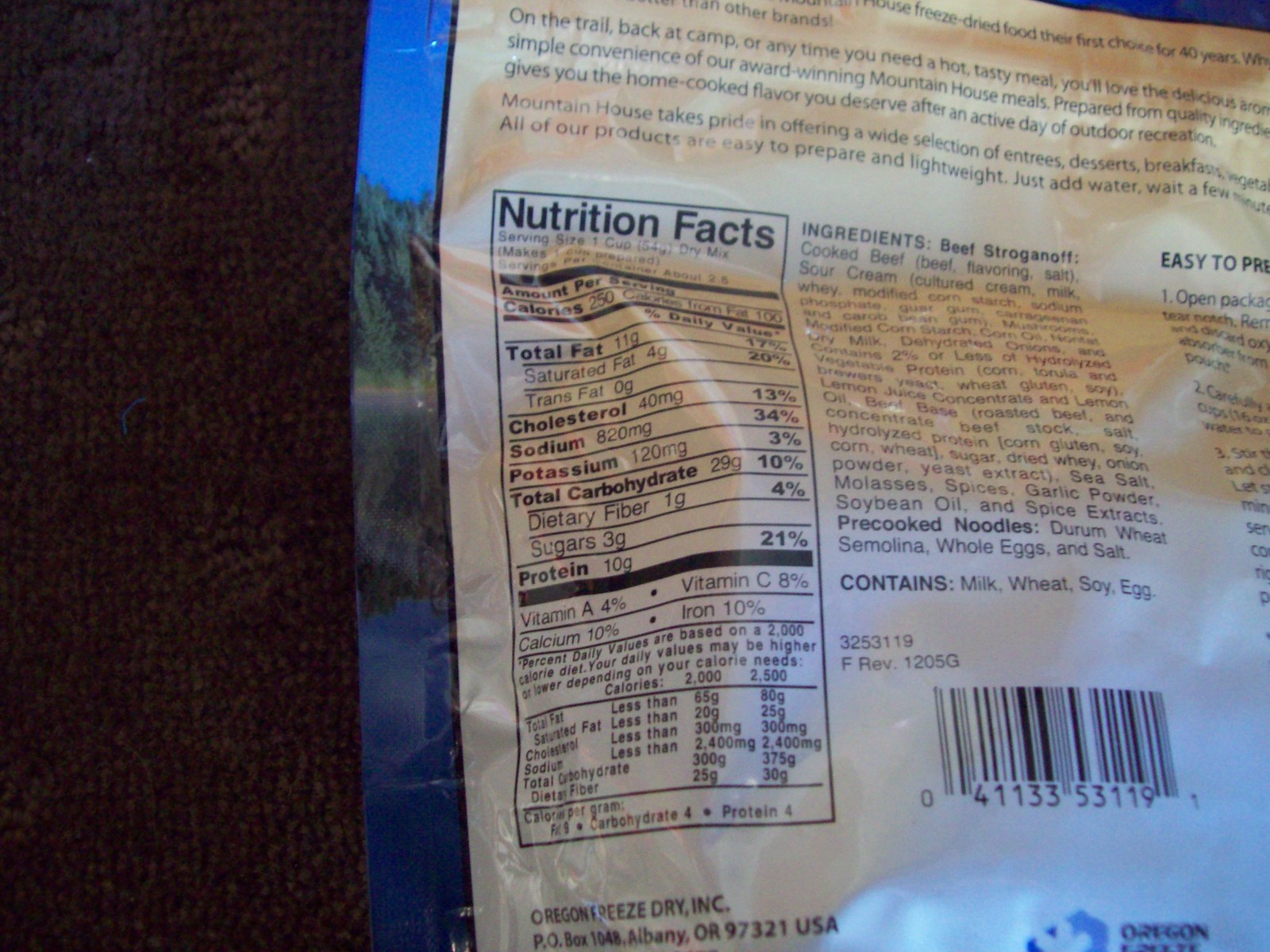The image captures the back side of a food package, prominently displaying the nutrition facts and partial product description. The top part of the description reads: "On the trail, back camp, or any time you need a hot tasty meal. You'll love the delicious [text cut off]. Simple, convenient, award-winning Mountain House meals prepared [text cut off]. Quality of ingredients [text cut off]. Gives you a home-cooked flavor. You deserve active outdoor recreation." The nutrition facts table provides detailed information such as calories, total fat, cholesterol, and other essential nutrients per serving. The ingredients list is also partially visible. 

The package appears to be made of plastic, complete with a barcode and preparation instructions along the edge. The design features what looks like a scenic mountain and lake illustration on the edge of the packaging. In the background, the item rests on what seems to be either a red or dark brown carpet.